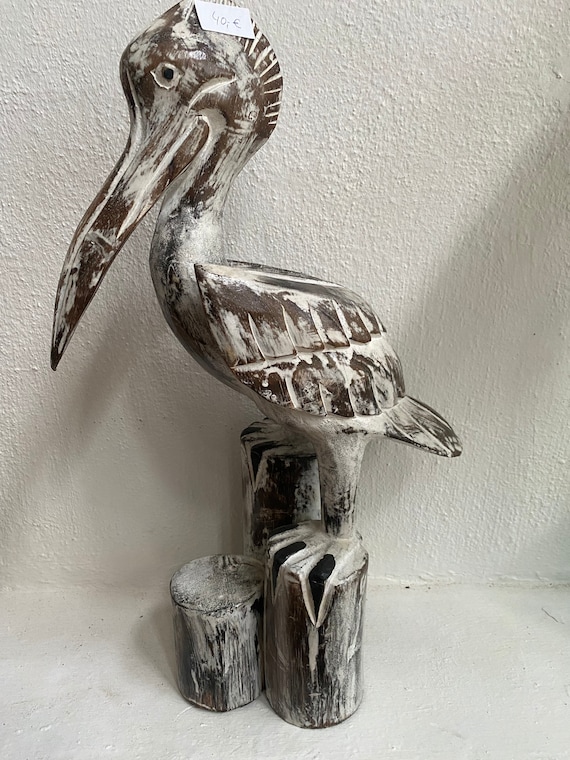This photograph showcases a rustic wood carving of a bird, possibly a stork or pelican, perched on three wooden stumps resembling posts found on a dock. The bird's legs straddle the two taller stumps at the back, while a shorter stump sits in front. The carving features striking details with textured feathers and a long beak, and the worn white paint reveals the natural wood beneath. The background consists of a white stucco wall, complementing the white floor or plaster countertop on which the carving stands, creating a stark contrast against the darker wood. A tag affixed to the bird displays the number "40," likely indicating a price in a foreign currency. The image, though in black and white, allows one to discern the rough texture of the surfaces and the nuanced light and dark areas of the sculpture.